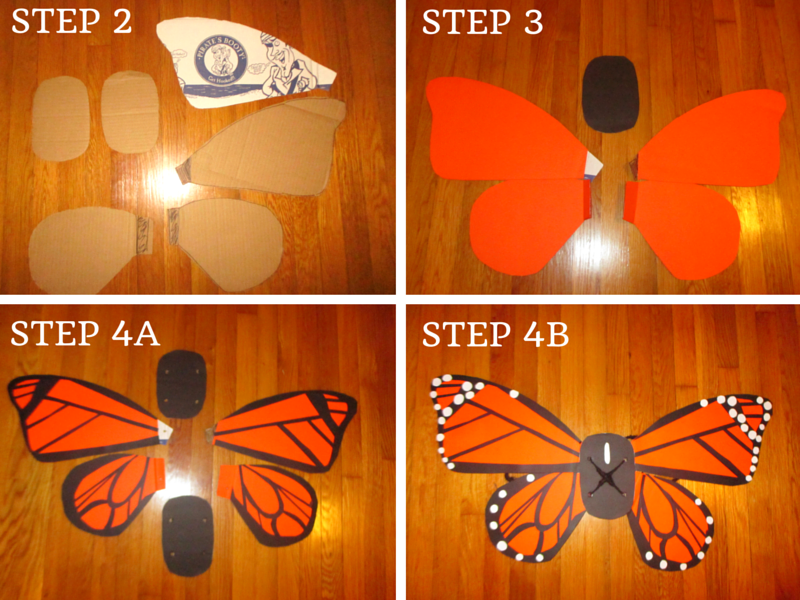The image is a detailed, step-by-step tutorial for making a craft butterfly using cardboard and colored materials, arranged in a two-by-two grid on a wooden surface. The first image, labeled "Step 2" in the upper left, shows pieces of cardboard cut in the shape of butterfly wings and a body. The second image, "Step 3" in the upper right, illustrates the painted cardboard sections, with the wings in bright orange and the body in black. The third image, marked "Step 4A" in the lower left, displays the butterfly with additional black designs on the orange wings, creating a more intricate pattern. The final image, "Step 4B" in the lower right, demonstrates the completed butterfly with white dots added to the wings for extra detail and a small decoration on the black body. The entire tutorial is clearly organized and shot from above, effectively guiding the viewer through the steps to create a decorative cardboard butterfly.